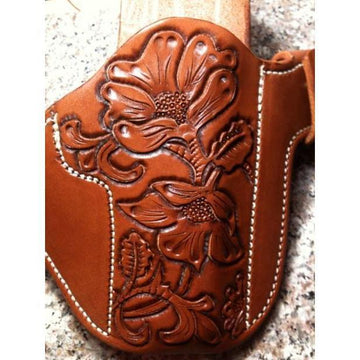The image displays a close-up view of a reddish-brown leather sheath, showcasing intricate craftsmanship. The sheath features a detailed pattern of engraved flowers that run vertically down the center, likely created using a leather stamping kit. The floral design extends from the top to the bottom of the sheath, flanked by solid leather areas on either side. These areas are accentuated by pronounced, thick white stitching that frames the floral pattern without overpowering it. Set against a bright, clear background, possibly a speckled counter or white surface, the sheath's rich color and detailed engravings are highlighted, making the image stand out vividly. The overall clarity and lighting of the image are excellent, ensuring every intricate detail of the leather and stitching is visible. The surrounding environment includes a wooden element, adding a touch of rustic charm to the composition.